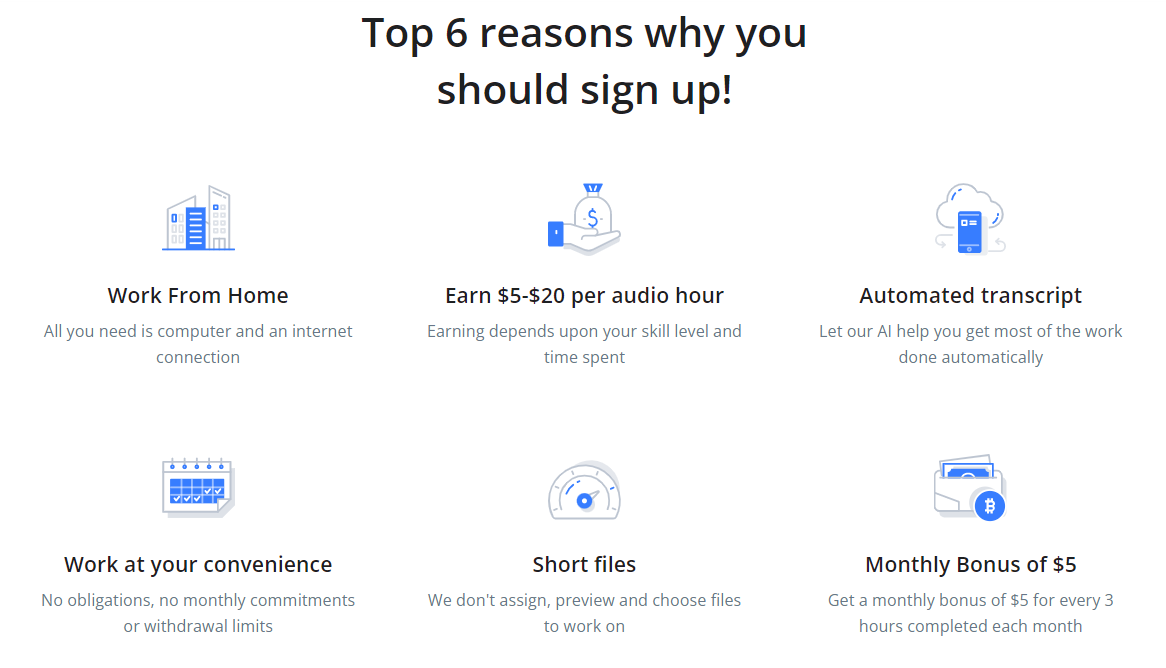The image is a screenshot of a web page detailing the top six reasons to sign up for a transcription service. The text is displayed in black letters and numbers. Below the heading, six options are organized in two rows of three.

In the top row:
1. **Work from Home:** This option explains that all you need is a computer and an internet connection.
2. **Earn $5 to $25 per Audio Hour:** It specifies that earnings depend on your skill level and the time you commit.
3. **Automated Transcripts:** An AI helps you automatically handle a significant portion of the work.

In the bottom row:
1. **Work at Your Convenience:** Highlighted benefits include no obligation, no monthly commitments, and no withdrawal limits.
2. **Short Files:** This note assures that you can preview and choose the files you wish to work on, implying that the files are manageable in length.
3. **Monthly Bonus:** You can receive a $5 bonus for every three hours of work completed each month.

Each point is accompanied by brief descriptions that emphasize the flexibility, potential earnings, technological assistance, user control, and additional incentives offered by the service.